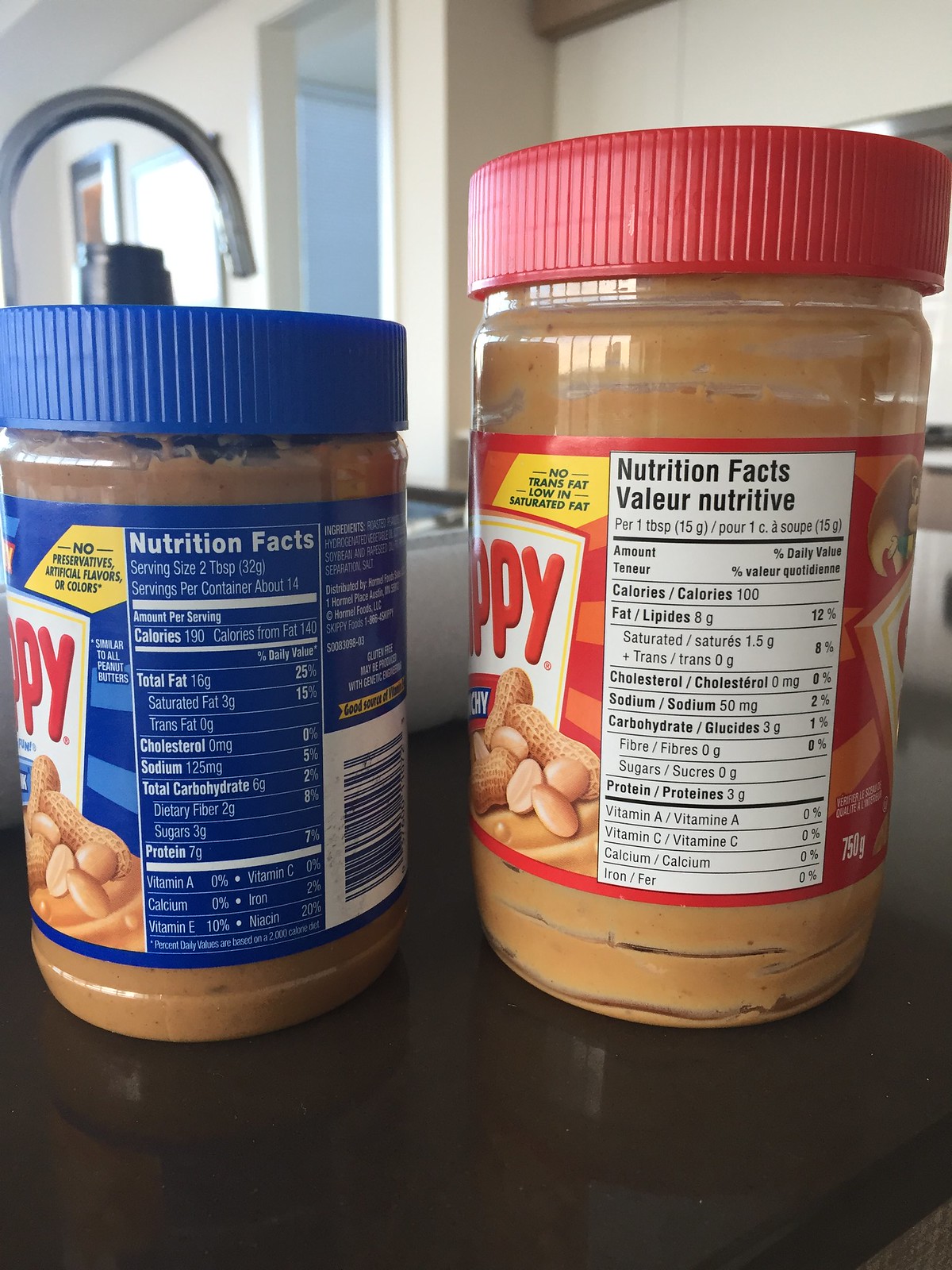The image depicts two jars of peanut butter in clear plastic containers showcasing the rich brown contents inside. On the left, a smaller jar is adorned with a blue lid and a matching blue label, while on the right, a slightly larger, taller jar features a red lid and a coordinating red label. Although the brand name is partially obscured, both labels end in "PP" or "PY," suggesting they are likely from the Skippy brand. The labels are decorated with an icon of several shelled and deshelled peanuts falling into a dab of peanut butter. The red-labeled jar prominently displays a yellow box with dark print stating "No Trans Fat, Low in Saturated Fat." Similarly, the blue-labeled jar features a small yellow section that reads "No Preservatives, Artificial Flavors, or Colors." Both jars rest on a nearly black countertop, with a light-colored wall and a kitchen faucet visible in the background, hinting at a cozy kitchen setting.